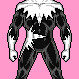The image is a small, square digital illustration against a uniform pink background, devoid of borders or text. It depicts a portion of a character, conceivably a digitally-generated superhero, from just above the knees to below the chest, excluding the face and lower legs. The character is rendered in a form-fitting, black, and gray armored outfit with distinct white accents. A notable feature is the white, pointed scarf-like design adorning the chest and shoulder area, resembling sun rays. The outfit includes a revealing slit at the waist, bordered with similarly pointed white fabric. The long sleeves extend slightly past the elbows, ending in white gloves, and both hands rest, fisted, at the sides of the thighs. Despite some blurred features, the character’s fit and muscular build is discernible. The absent head and lower legs emphasize the central portion of the body, highlighting the intricate costume details against the stark pink background.